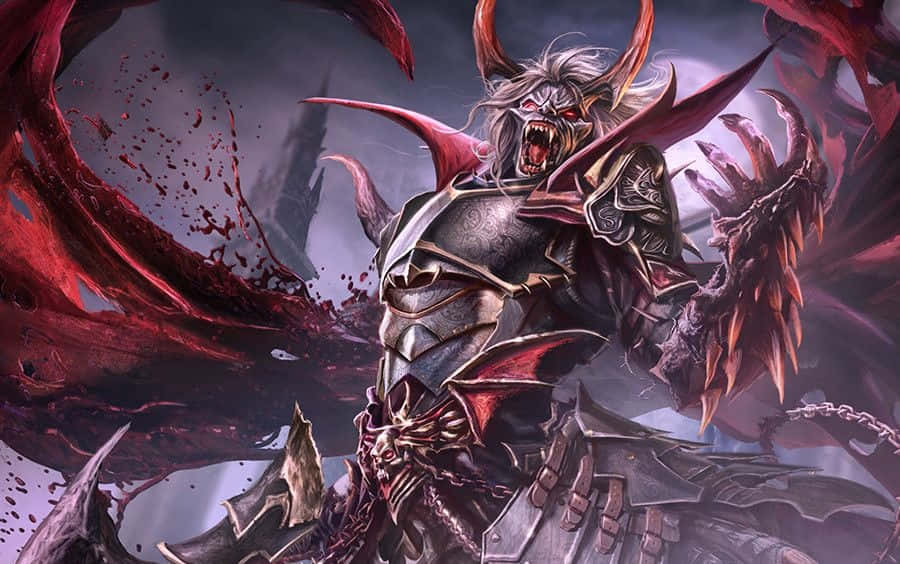This highly detailed and vividly colored computer-generated image showcases an imposing video game character, designed in a menacing style typical of supernatural antagonists. The character features a terrifying demon-like face adorned with huge animal-like fangs, glowing red eyes, and deeply wrinkled skin. Its long hair, which appears either gray or blonde, cascades around its face, accentuated by two red horns protruding from its head. 

The character's robust frame is encased in formidable body armor, complete with metal shoulder pads and arm plating, and it sports clawed, demon-like hands with massive fingernail-like claws. Additional spikes jut menacingly from its arms and back. A skull adorns the belt, adding to the ominous aesthetic, and chains are visible in the background, hinting at a possibly sinister confinement.

Behind the monstrous figure, an intense scene unfolds—red liquid that resembles blood flies and spews through the air. Dominating the background is a towering castle-like structure with an extraordinarily tall steeple. The scene is bathed in the eerie light of a full moon, whose shadowy presence adds an extra layer of foreboding. This detailed and disturbing image appears to be taken from a fighting or fantasy video game, with the character poised for battle, exuding an aura of rage and ferocity.